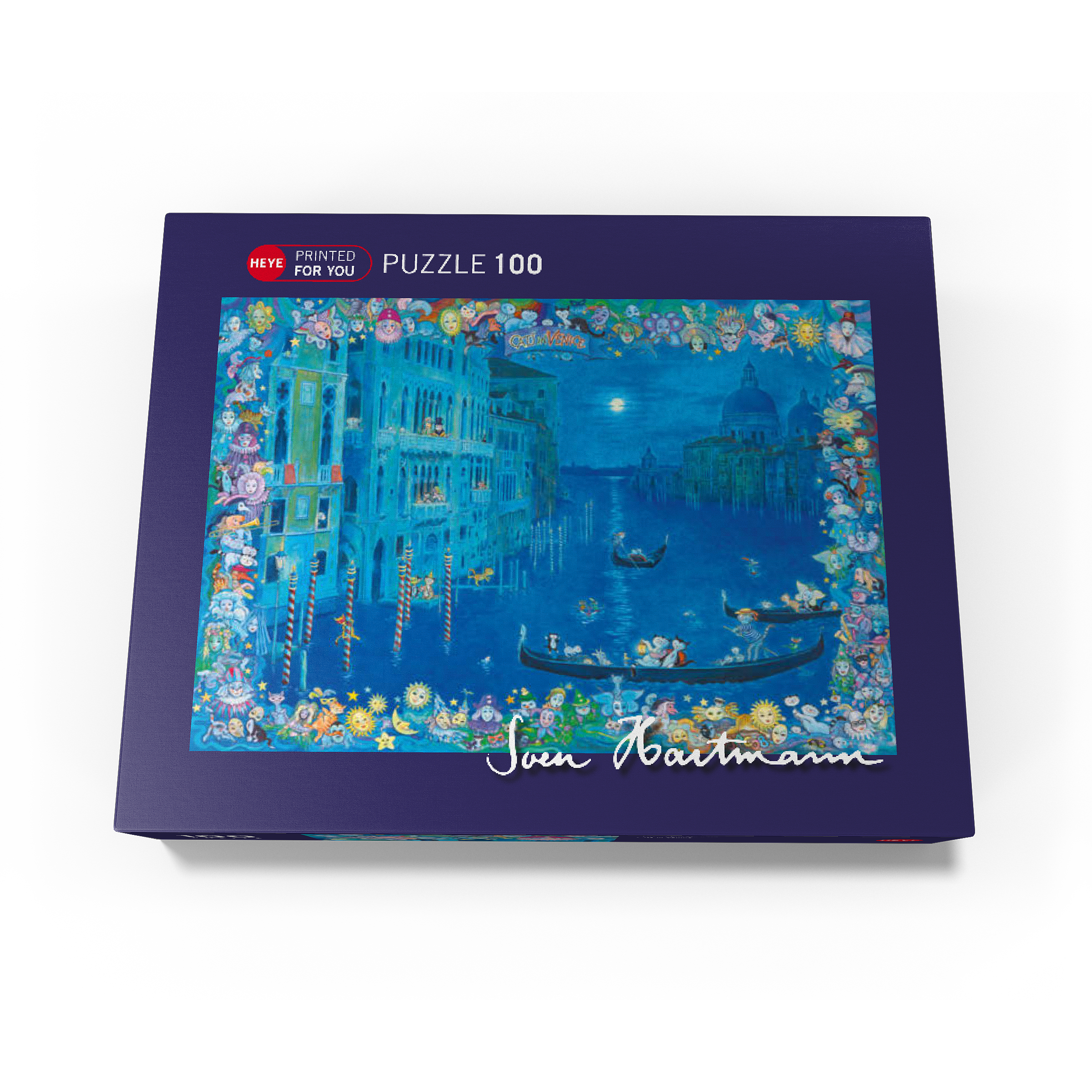This is an image of a rectangular jigsaw puzzle box cover with a dark purple background. In the upper left-hand corner, there is a red circle with white letters spelling "H-E-Y-E." To its right, a red oval outline contains the text "Printed for you" in white. Next to this, in white letters, it reads "Puzzle 100." The center of the box features an illustration of a nighttime canal scene, reminiscent of Venice, dominated by bluish hues. The scene includes three gondolas floating on the water, filled with whimsical characters like cats and flowers with faces. On both sides of the canal are several tall buildings; on the left, colorful barbershop-like striped poles stand out, while on the right, there is a distinctive building with a dome and tower. The moon is visible in the sky, casting a reflection on the canal. Surrounding the main illustration is a vibrant border adorned with various bright designs, including suns with faces, clowns, stars, and moons. The name of the artist, Sven Hartmann, is also displayed.